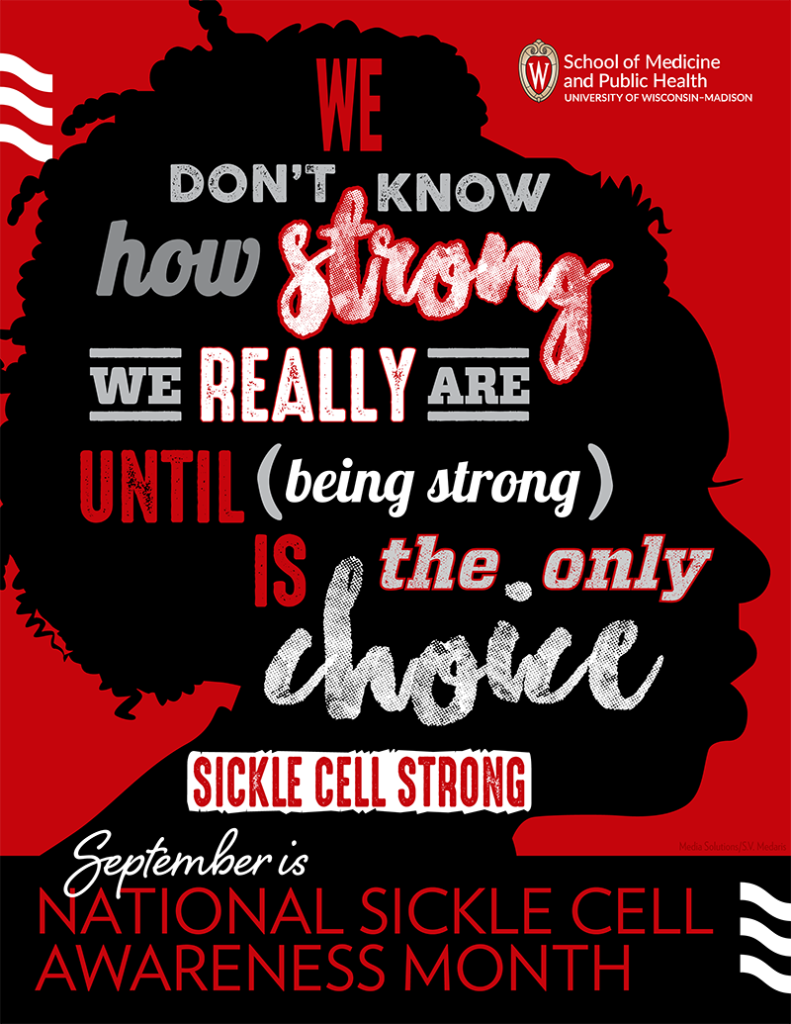This image from the School of Medicine and Public Health at the University of Wisconsin-Madison prominently features a powerful and compelling poster dedicated to National Sickle Cell Awareness Month. Dominated by a solid red background, the centerpiece is a striking black silhouette of a black woman in profile, her head and hair distinctly outlined. Within the silhouette, layered in a mix of red, gray, and white text, the inspirational message, "We don't know how strong we really are until being strong is the only choice," is emblazoned, emphasizing the theme of resilience. Just below the profile, "Sickle cell strong" is highlighted in red text inside a white box, further emphasizing the focus on strength in the face of adversity. Towards the bottom, a bold black bar stretches across the poster, featuring the cursive white text, "September is," followed by large, thin red letters declaring, "National Sickle Cell Awareness Month," to remind viewers of the significance of the month. The overall design and color scheme powerfully underscore the themes of strength and awareness.